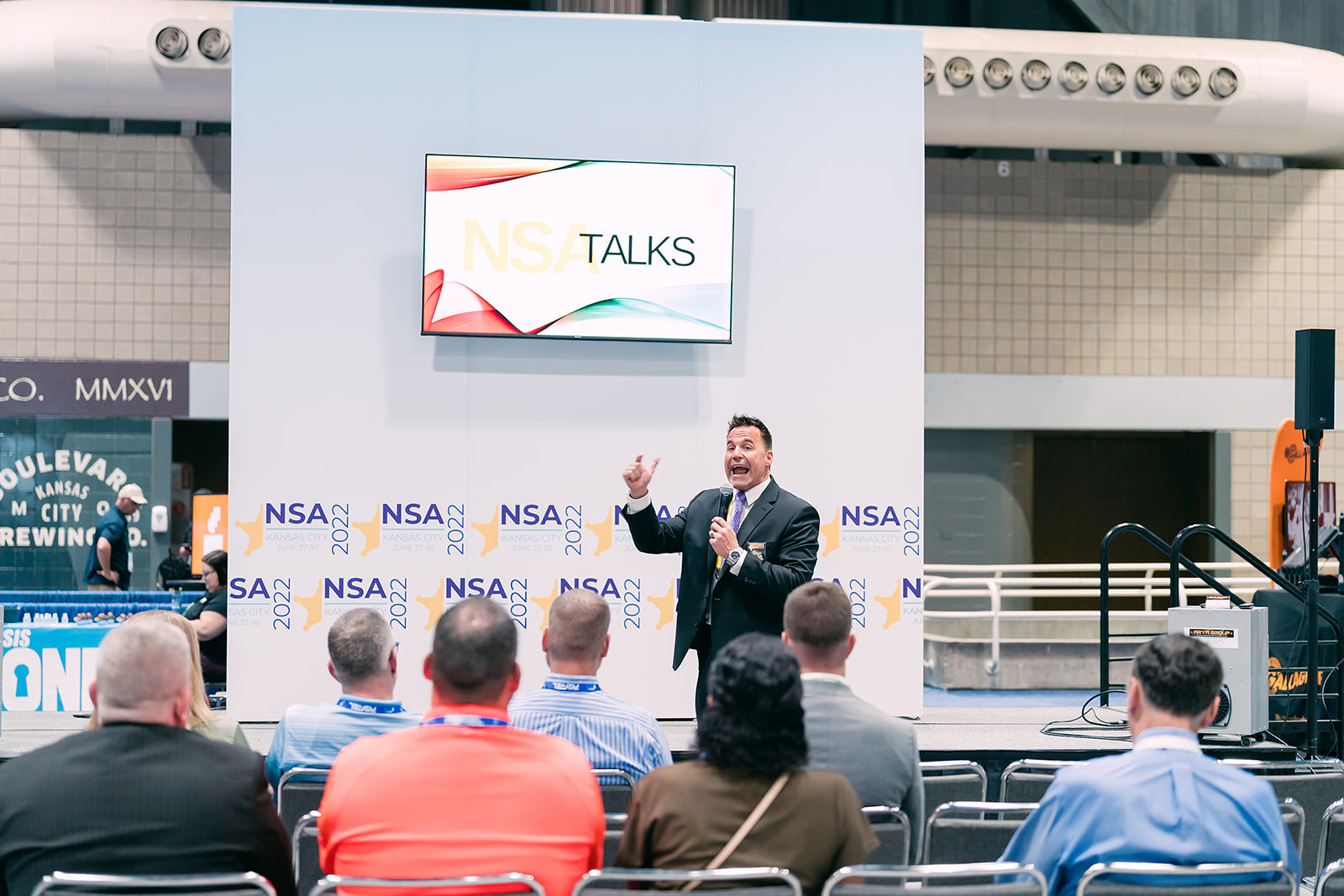The image is an indoor rectangular photograph, taken from the audience's perspective, capturing a speaker on a small stage. The gentleman on stage, dressed in a dark suit jacket, a white shirt, and a purple tie, holds a microphone in his left hand while his right hand is extended outward with his thumb and forefinger spread apart. He appears to be addressing the audience, given his open mouth and expressive gesture. Behind him, a large billboard or poster board prominently displays "NSA talks" at the top and is bordered at the bottom with repeated logos reading "NSA 2022" accompanied by several stars. In the foreground, seven audience members, both men and women, are seated on metal-framed chairs. Most of them are wearing lanyards, primarily blue with white print, although some have different colors such as white or black. They are attentively watching the speaker.